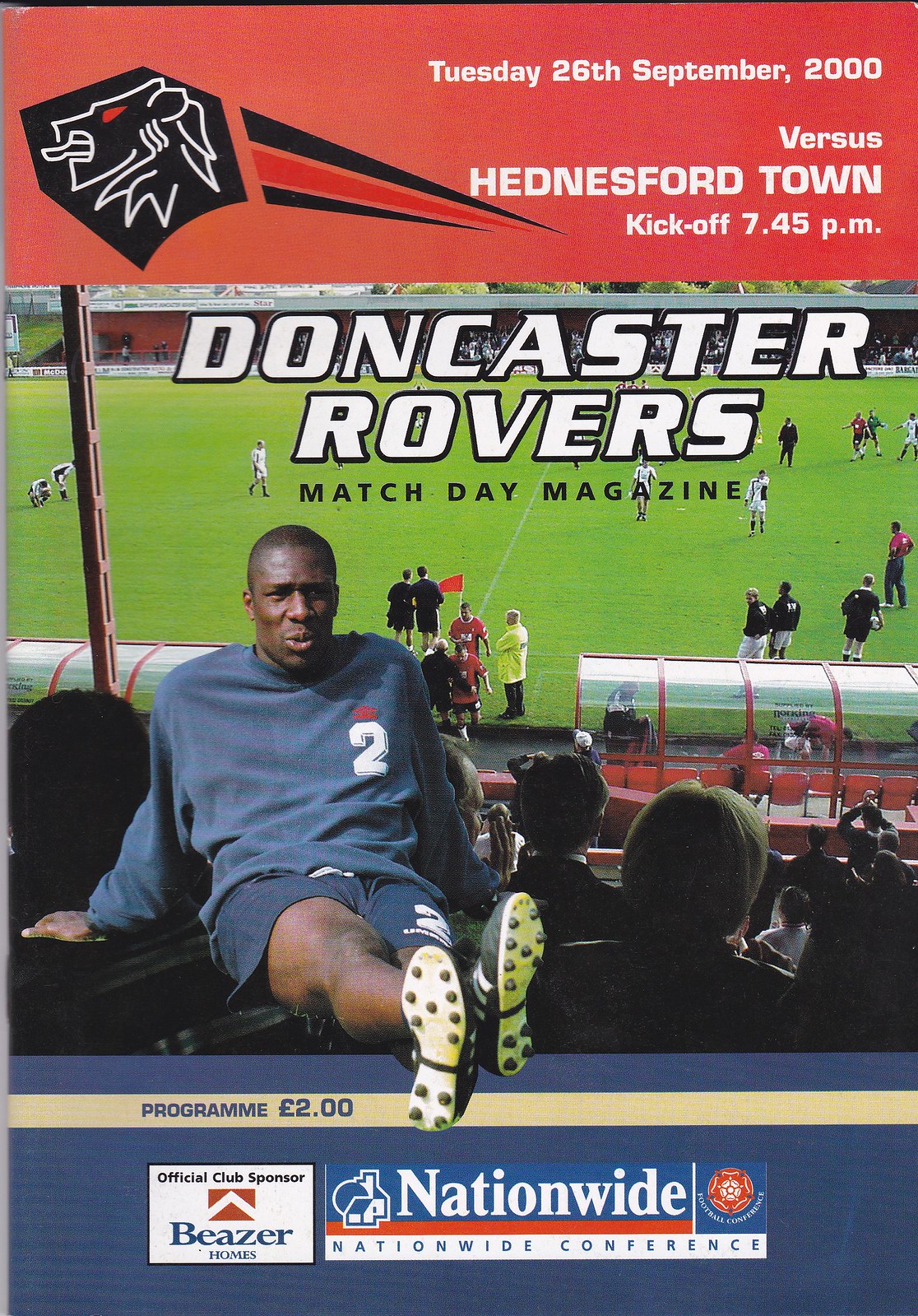The image is a scan of a Doncaster Rovers Match Day magazine for a game held on Tuesday, 26 September 2000, against Hednesford Town, with kickoff scheduled for 7:45 p.m. The magazine cover has a prominent red background at the top, featuring a black and white lion's head logo. Below the date and match details, there's a photo showing a soccer field with players in action and spectators in the stands. Superimposed atop this scene is a casually dressed player, wearing the number 2 jersey, sitting cross-legged and making a playful expression. The title "Doncaster Rovers Match Day Magazine" is displayed above the image. At the bottom, a blue border contains a white banner, which states "Program £2.00," alongside logos for the official club sponsor, Beezer Homes, and the Nationwide Conference.